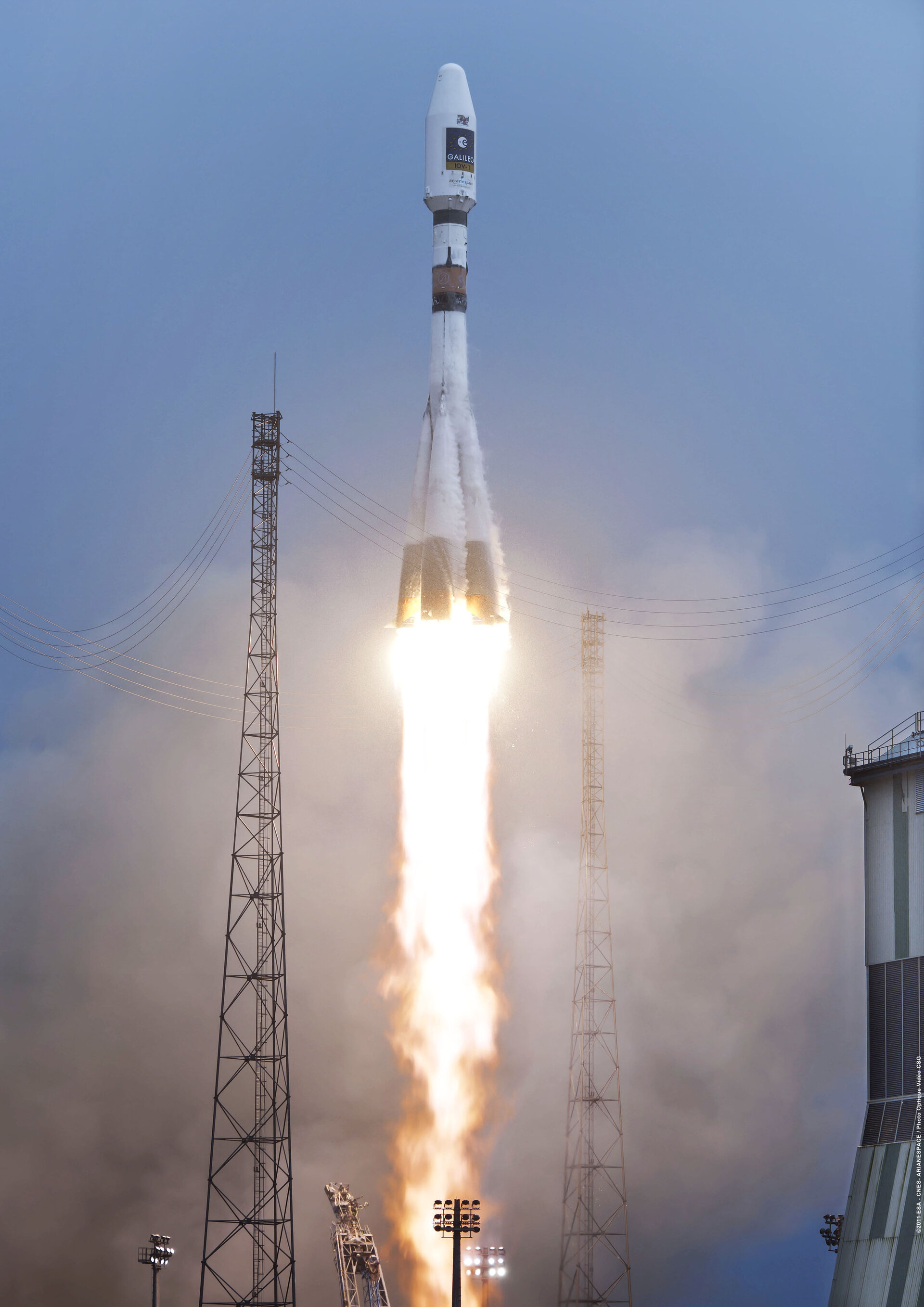This image captures an active rocket launch under clear blue skies, showcasing a white rocket adorned with black and brown accents. The rocket, potentially intended for launching a satellite or unmanned mission rather than a crewed shuttle, displays distinct segments that merge as it ascends. Below the ascending rocket, an intense stream of flames propels it skyward, surrounded by a large plume of white and gray smoke. Two tall power line towers flank the sides of the scene, with an observation tower visible on the right. Bright stadium-like lighting apparatuses illuminate the vehicle, highlighting the stabilizing structures now released and leaned back following lift-off. The rocket, already several stories high—likely around ten stories at this point—is in the midst of its powerful ascent into the atmosphere.